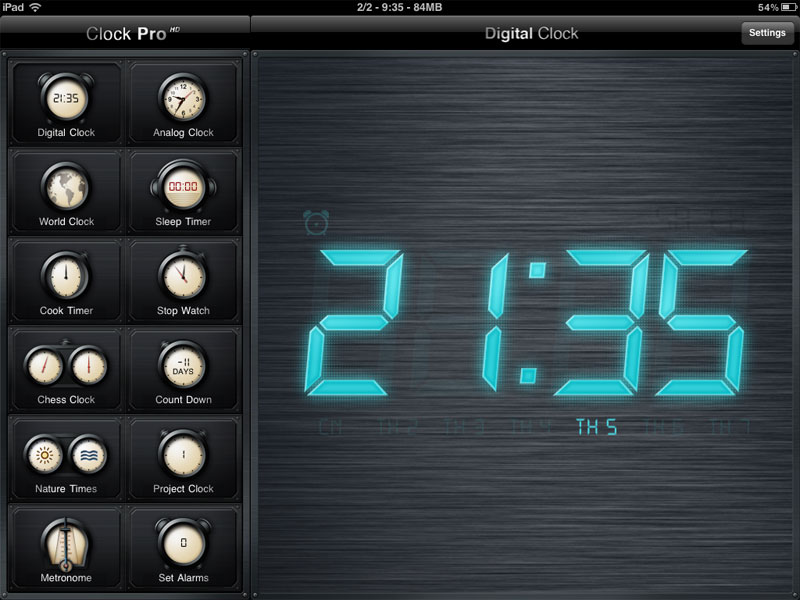Here's a cleaned-up and detailed caption for the image:

A zoomed-in shot of the black housing of a multifunction digital clock. On the right-hand side of the image, a line-textured black panel prominently displays aqua blue lettering that reads "21:35 PH5." Directly above this panel, the words "Digital Clock" are printed in white on the housing. On the left-hand side, the heading "Clock Pro" is also written in white lettering. Beneath this heading, there are two columns of several buttons arranged vertically along the left side of the image. These buttons are labeled sequentially from top to bottom as follows: Digital Clock, Analog Clock, World Clock, Sleep Timer, Cook Timer, Stopwatch, Chess Clock, Countdown, Nature Timer, Project Clock, Metronome, and Set Alarm.